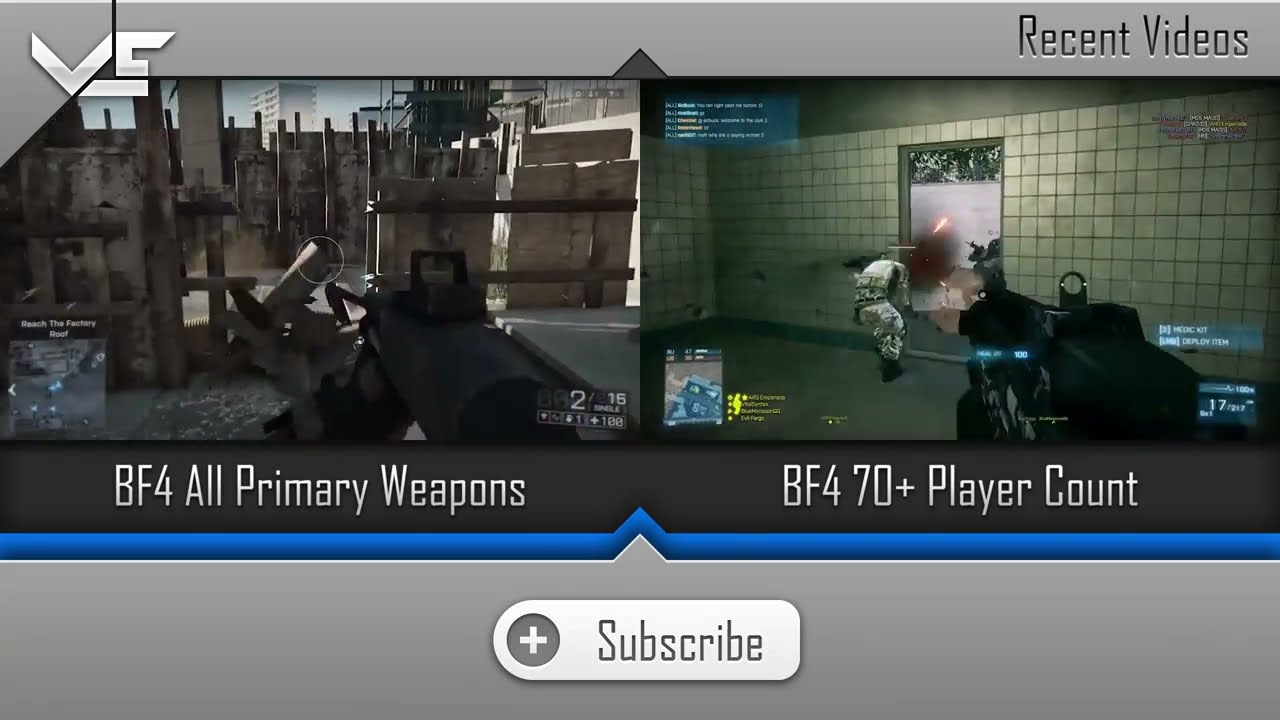The image is divided into two distinct sections, both showcasing still shots from a video game. On the left, labeled "BF4 All Primary Weapons" in white text, is a snowy yard scene with cannon-like weapons. Wooden boards are propped against a wooden fence, resembling makeshift practice shot walls. The top-left corner features a logo that appears to be "VCN" or "VC." The border is steel gray, with the bottom containing an oval-shaped subscription button outlined in white and gray, with a white plus sign on the left side.

On the right side, titled "BF4 70+ Player Count" in white text, we see a soldier inside a building with white tiled walls, standing in front of a doorway with visible bullet holes. Explosions are occurring outside, and the soldier appears to be in a bending position, possibly after being shot. Through the doorway, a gun is pointed outside at unseen enemy soldiers. The top-right corner includes the text "Recent Videos." The overall setup suggests a detailed look into different scenarios within the game.